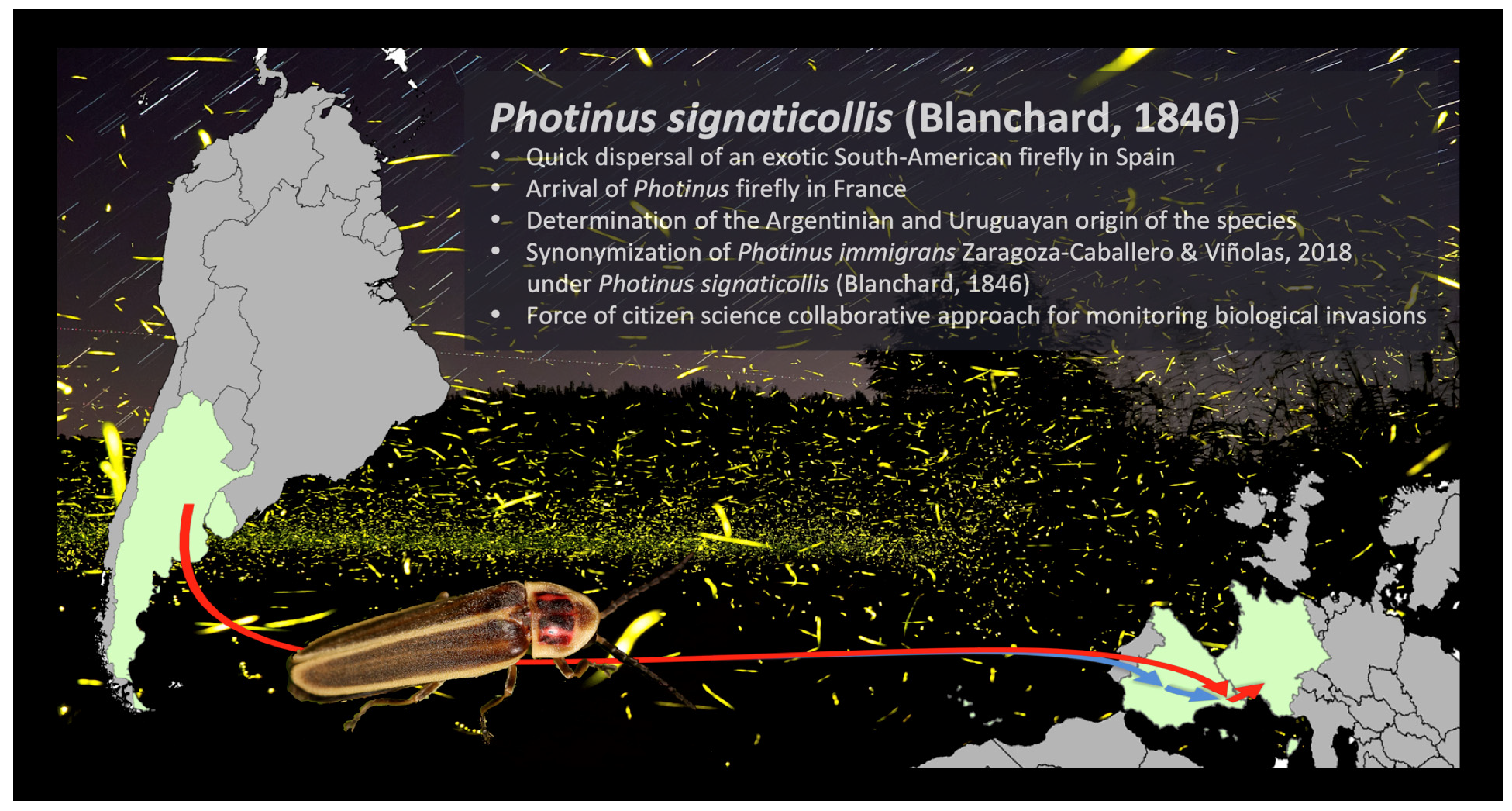This poster image features a detailed graphic illustrating the spread of an exotic South American firefly species. On the left side of the image, there is a grey map of South America marked with black country borders. Argentina is highlighted in light green. From Argentina, a red line extends to the right, passing over a cockroach illustration, and culminates in a map of Europe on the right side, with Spain similarly highlighted in green.

At the top right of the image, the title "Photinus Cygnaticolus, Blanchard, 1846" is prominently displayed in white text against a dark grey background that transitions to black at the bottom. Below the title, a list of five bullet points provides key information:

1. Quick dispersal of an exotic South American firefly in Spain.
2. Arrival of the Photinus firefly in France.
3. Determination of the Argentinian and Uruguayan origin of the species.
4. Synonymization of Photinus emigrans Zaragoza-Caballero and Vinolas, 2018 under Photinus Cygnaticolus, Blanchard, 1846.
5. Force of citizen science collaborative approach for monitoring biological invasions.

The entire background is sprinkled with small yellow lines or dots, resembling fireflies. This comprehensive visual and textual presentation underscores the firefly's migration from Argentina to Europe, supported by insights into the species’ origins and the role of collaborative citizen science in tracking biological invasions.